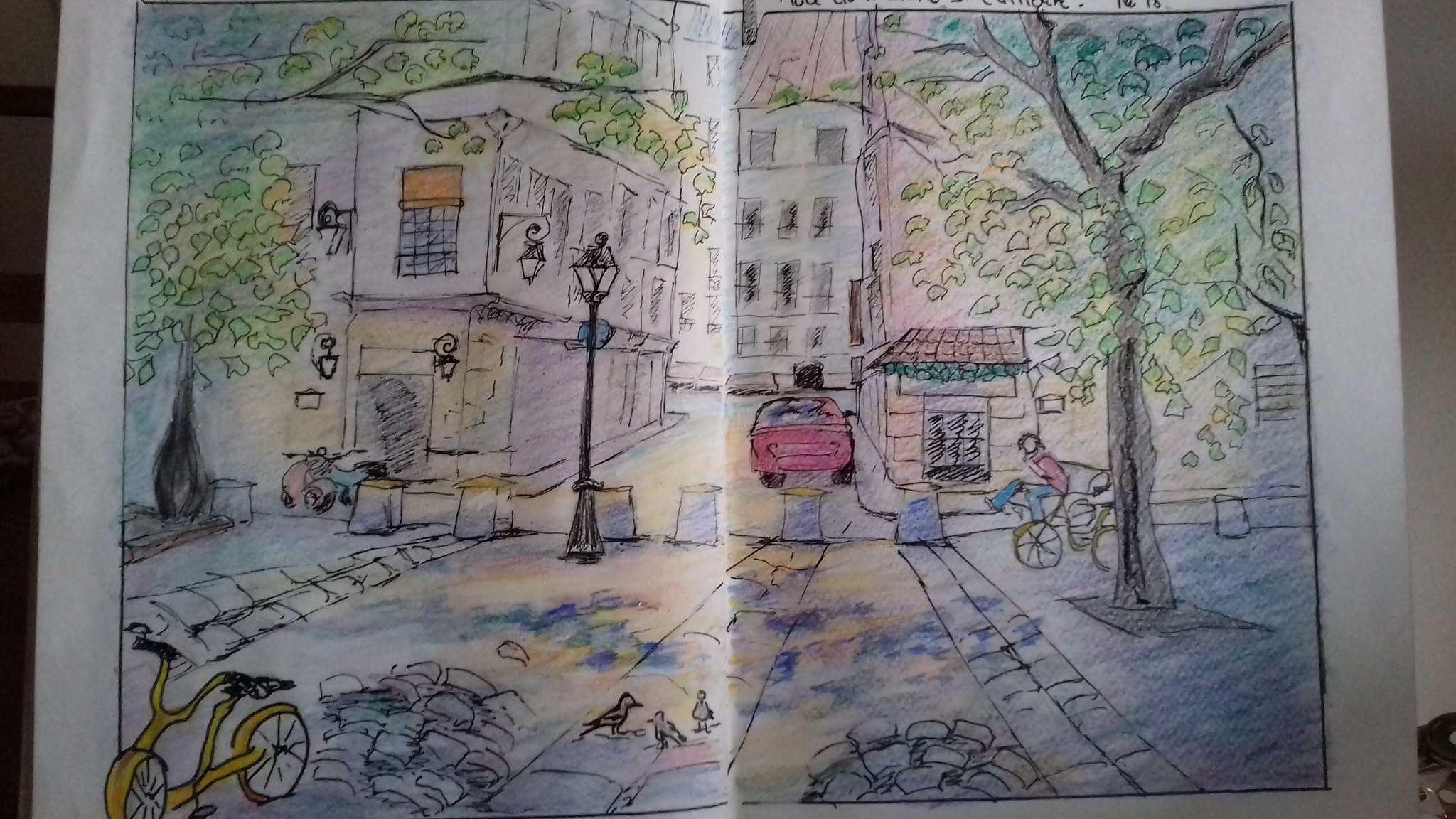The image features a detailed drawing on a large, folded white sheet of paper, resembling a city street view. At the center of the composition, a road runs upwards towards a row of buildings, framed by trees with brown trunks and leafy canopies—the left tree sporting lime-colored leaves and the right tree, a lighter green hue. 

On the bottom left-hand corner, a yellow bicycle rests near a cluster of stones. Midway on the street stands a trio of birds, adjacent to additional stones. Heading up the street, a red car moves towards the background, adding a splash of vibrant color among the predominantly shaded, light brown and white buildings. On the right side of the image, another person sits on a bench next to a yellow bicycle, blending into a scene punctuated by tall black streetlights with lantern-like tops. 

A unique element of this artistic depiction is its method of coloring: although the scenes of grass and paths around the urban setting don't adhere to typical green shades, using instead a bluish-yellow palette, the foliage retains a delicate mix of lime and light green. The artistry and attention to minute details like the blue motorbike next to the left-hand tree and the person in a red shirt and blue jeans, create a lively yet serene neighborhood block capturing the essence of city life.